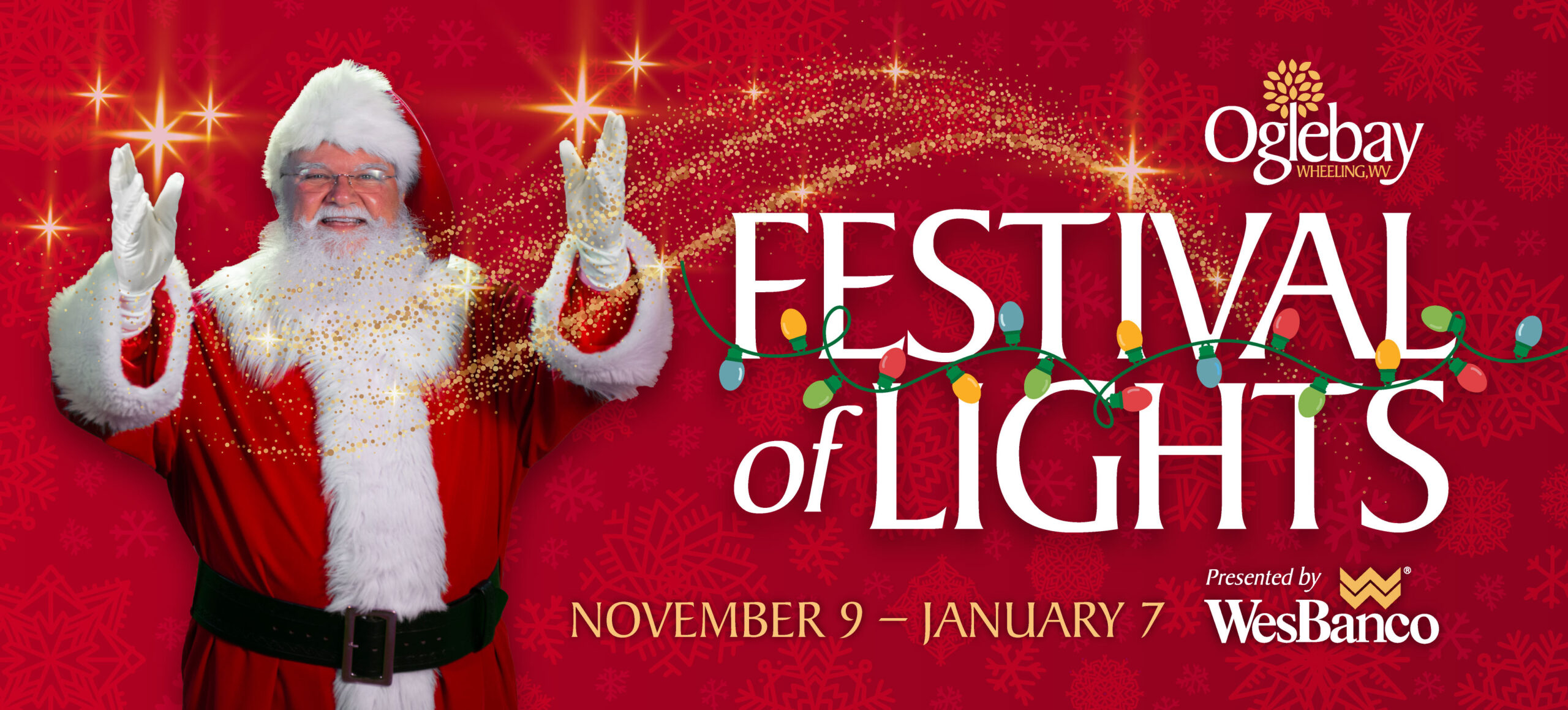This promotional poster, professionally crafted and horizontally rectangular, features a festive and vividly detailed scene set against a rich red background adorned with subtle watermarked snowflakes. The left side prominently showcases Santa Claus in his full Christmas regalia—bright red suit with white fur trim, matching hat, white gloves, black belt, glasses, and a full white beard. He raises his hands, smiling broadly, with digital sparkles emanating from his fingertips, adding a touch of magic. 

On the upper right corner, the poster displays the text "Oglebay Festival of Lights" in bold white letters, with colorful cartoon Christmas lights woven between the words "Festival" and "Lights." Below that, the dates "November 9 – January 7" indicate the event's duration, followed by the note "Presented by WesBanco," denoting the event sponsor. The overall impression is one of holiday excitement, inviting families to enjoy the seasonal light show extravaganza in Wheeling, West Virginia.